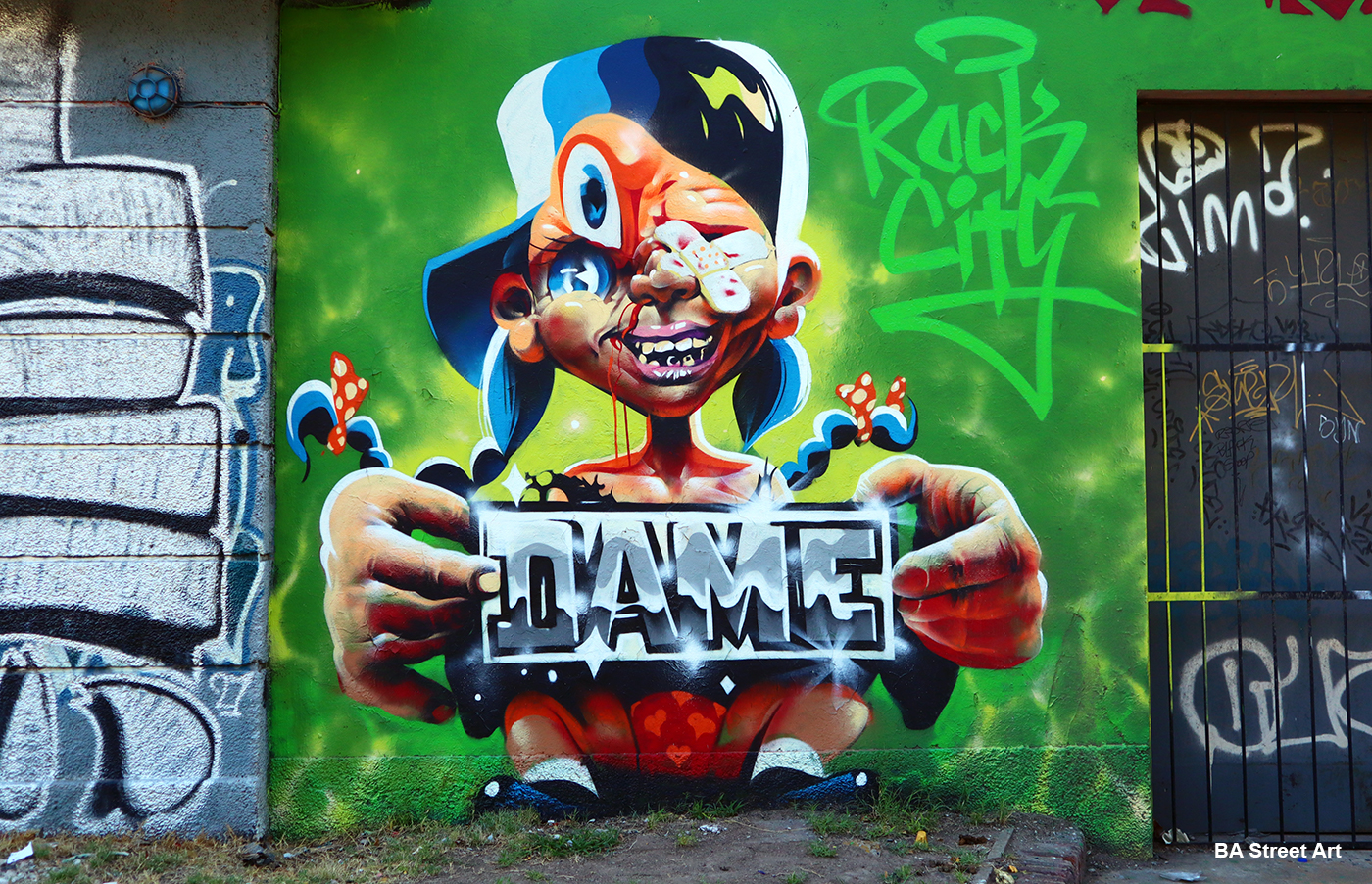The image features an intricate piece of street art on the side of a building, vividly showcasing a character with a blend of vibrant colors. Dominating the green wall, the central figure is a peculiar representation of a woman adorned in detailed graffiti. She wears a multi-shaded blue baseball cap cocked to the side and sports braided pigtails tied with red and pink polka-dotted hair ties. Her exaggeratedly large hands hold a sparkly sign that reads "Dame," which covers most of her body. Below, her thick legs and feet are painted to align perfectly with the ground, making it appear as if she is seated against the wall in reality. Her face is grotesque yet meticulously detailed, with a broad smile, damaged bottom teeth, a single prominent eye, another eye covered with band-aids, and a third eye in a different style, symbolizing a deeper commentary. Additional graffiti adorns the setting, including the tags "Rack City" above and "BA Street Art" in the bottom right corner. To the left, a gray cement wall with partially visible graffiti peeks into the frame, while to the right, a barred door also marked with graffiti completes the urban tableau. The entire scene, set against a rainbow-like spectrum of colors, exudes a juxtaposition of raw, gritty street life with an element of satirical sophistication.